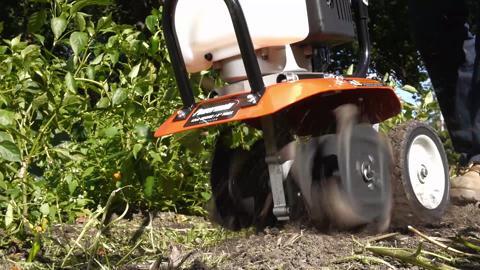The image showcases a close-up of a subcompact, gas-powered tiller in operation, designed for breaking up soil for cultivation and planting. The tiller features a small engine reminiscent of those found on weed trimmers, encased in a white metallic cover at the top center. A black exhaust hose is visible, leading from the engine, and a horizontal black handle or bar at the front aids in maneuvering. There's also a small black card likely indicating the machine's specifications.

The front section of the tiller includes two rotating cultivating discs or tines, slightly blurred to indicate motion, used to dig into and turn over the soil. These are partially shielded by an orange fender to protect the motor from dirt. The tiller is equipped with two front wheels that appear to aid in cutting, and two back wheels with more pronounced treads for stability and movement across the ground.

In the backdrop, the scene divides into two contrasting areas: on the left, a dense cluster of green foliage, and on the right, recently tilled ground with sticks and debris, showcasing the tiller's impact. The photograph is tightly cropped, focusing on the lower section of the tiller, emphasizing its functional parts in action on a patch of bare, flattened grass.